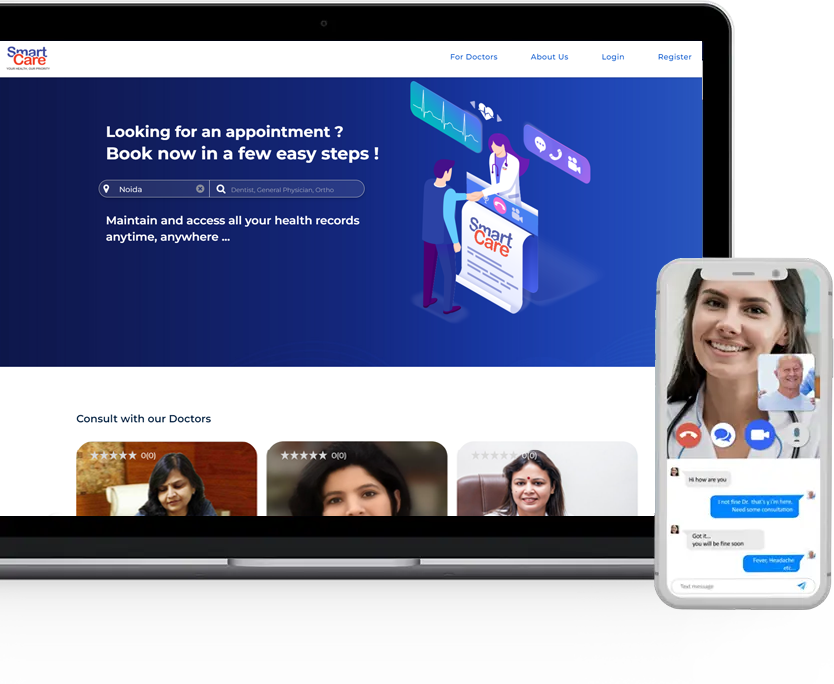Here's a cleaned-up and detailed caption for the described image:

---

A sleek laptop screen displays a website branded as "SmartCare." The header features a white bar, with the word "Smart" in bold blue text and the word "Care" in bold red text slightly overlapping. On the right side of the header, there are navigational links written in blue text: "For Doctors," "About Us," "Login," and "Register."

Below the header, a large blue graphic area showcases a cartoon-style illustration of a person shaking hands with an individual wearing a lab coat, implying a doctor-patient interaction. Above this illustration, various icons are depicted, representing the services offered.

To the left of the illustration, white text reads, "Looking for an appointment?" followed by, "Book now in a few easy steps!" Additionally, there's a search bar and clickable icon labeled "Nodia."

Further down, the website emphasizes, "Maintain and access all your health records anytime, anywhere," with visuals showing consultations with three different female doctors.

On the right side of the page, an image of a smartphone is displayed, depicting a chat-like interface where a user is having a telehealth conversation with one of the doctors. The messages at the bottom indicate real-time communication, simulating either a phone conversation or text-based messaging.